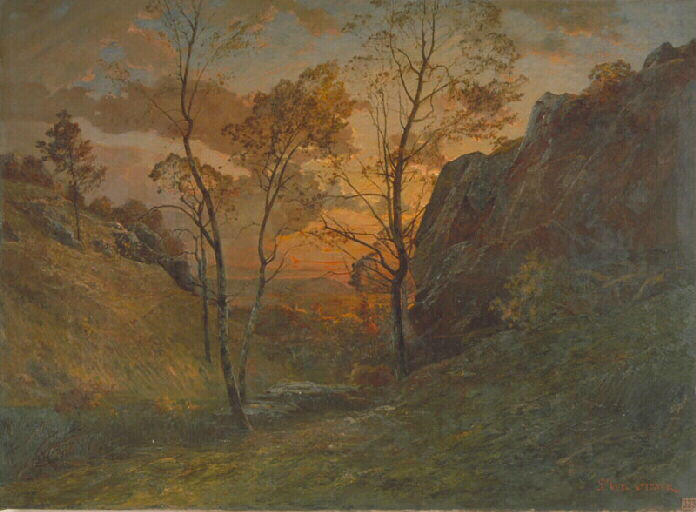The image captures a serene evening landscape, showcasing a blend of natural features under a dramatic sky. Dominating the right side is a tall, imposing rock barrier, possibly a mountainside, painted in shades of brown and gray. Centered in the scene are three tall, slender tree trunks with sparse yellowish leaves, standing prominently amidst a verdant stretch of grass and smaller trees. On the left, a gentle hillside slopes upward, adorned with another tree. The sky above is a captivating mix of hues—orange, reddish-pink, gray, blue, and mustard yellow—indicative of a sunset casting its shadowy touch over the clouds. The atmosphere is hazy, with a grayish-blue color dominating. Despite the detailed depiction, there are faded areas adding to the scene's mystique. No people or animals are present, maintaining an undisturbed, tranquil aura. Notably, in the bottom right corner, there's a light red or orange inscription that appears to be a signature. The overall palette comprises gray, green, and brown, emphasizing the natural and earthy tones of the landscape.